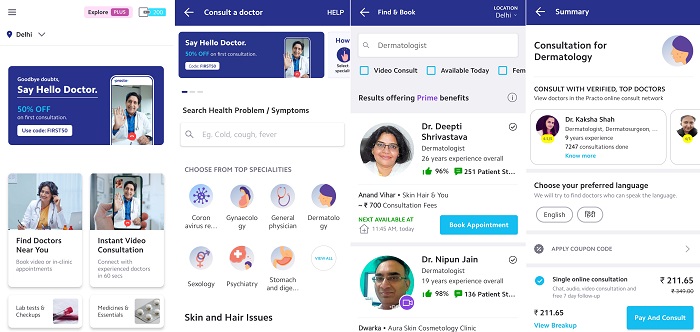The image showcases a telemedicine platform prominently featuring healthcare services and consultation options. The webpage is led by a headline, "Consult a Doctor" and offers functionalities like booking appointments, accessing summaries, and locating services, though these navigation options appear small and are situated at the top.

At the forefront, there is a vibrant section with the greeting "Say hello to the doctor," accompanied by a cheerful image of a female doctor waving. The platform advertises a 50% discount code for services.

Below, it encourages users to "Find a Doctor Near You" and offers "Instant Video Consultation." The second column reiterates the "Say hello to the doctor" message, showing the same image of the doctor waving. There's an interactive question bar for users to input symptoms, and a section to choose from top specialties such as skin and hair issues, and dermatology. 

Highlighted is an offering for video consultation available today, promoting results with prime benefits. Featured is a dermatologist with 26 years of experience displayed alongside another dermatologist with 19 years of experience. Both profiles include patient ratings, the number of patients seen, and consultation details.

The page also presents an option to choose your preferred language (default being English) for consultations. Lastly, it provides pricing information for a single office consultation, listed at $211.65, with an option to pay and proceed with the consultation.